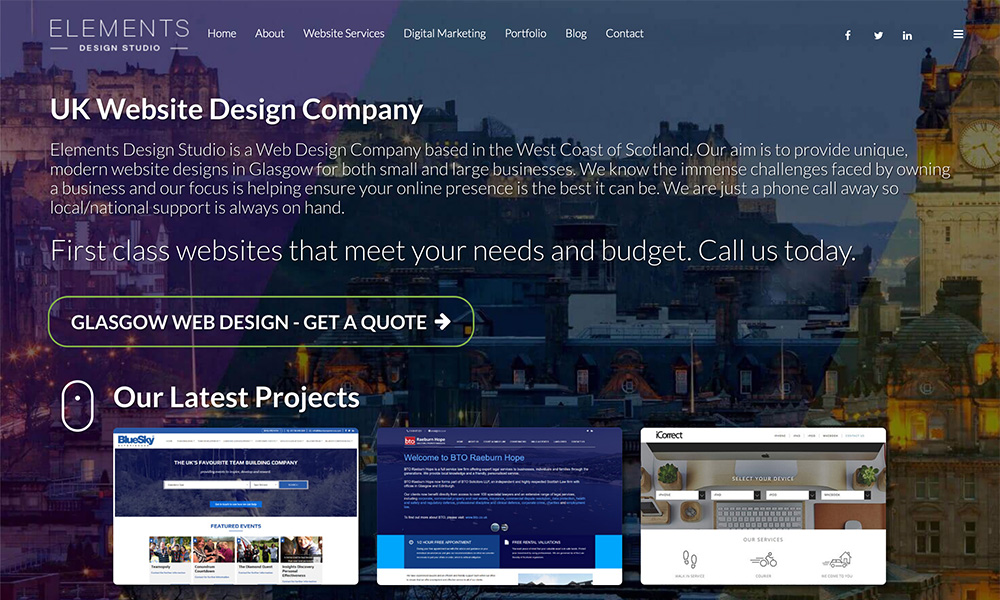Screenshot of a professional web design company's homepage.

In the upper left section of the page, there is a navigation menu with the following links: Elements, Design Studio, Home, About, Website Services, Digital Marketing, Portfolio, Blog, and Contact. Positioned in the upper right, there are icons for social media platforms—Facebook, Twitter, and LinkedIn—followed by a hamburger menu icon represented by three horizontal lines.

The primary text block introduces "Elements, Design Studio," a web design company based on the west coast of Scotland. The text emphasizes the company's mission to deliver unique, modern website designs tailored for both small and large businesses in Glasgow. The company acknowledges the challenges of running a business and aims to enhance clients' online presence through their local and national support services. 

Prominently displayed in larger text is a call-to-action: "First-class websites that meet your needs and budget. Call us today." Beneath this is a large button labeled "Glasgow web design," with an option to "Get a quote."

The background image of the webpage features a city view of Glasgow at night, likely showcasing famous landmarks of the city.

At the bottom of the screen, there's a section titled "Our latest projects," displaying small thumbnails of various web pages designed by the company. The featured projects vary in their design focus, with some being text-heavy and others image-heavy.